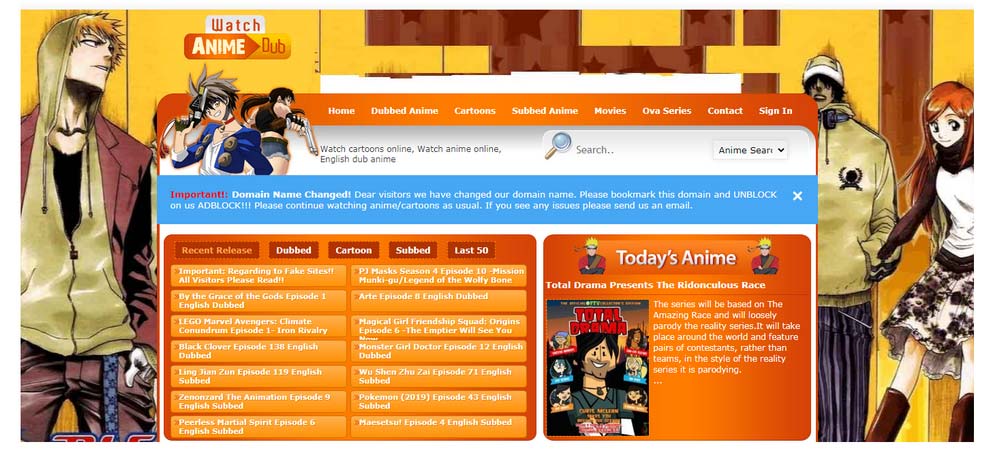A detailed description of an anime-themed website features a vibrant and intricate layout. The background prominently displays various anime characters. The color scheme includes a substantial yellow section that covers about one-third of the page, transitioning into a gradient of brown adorned with dark brown stars. This pattern repeats with alternating strips of yellow and brown, culminating in a vertical column on the right side.

On the right side of the page, there's a prominently featured anime character, positioned chest-forward with a slight head tilt to the right. This character has blonde hair and wears a green hoodie over a black shirt, layered with a red shirt on top. The ensemble is completed with red pants and a blue belt that hangs down.

On the left side, a female anime character with red shoulder-length hair is depicted. She wears a white shirt with red sleeves, paired with a black and white skirt and brown boots. Adjacent to her stands another anime character adorned in a hat and sporting brown hair. This character wears a yellowish-brown shirt combined with blue and black, or possibly purple and black, striped pants.

To the immediate right of the female character in white, a white tab with the word "WATCH" in red is visible. Below it, in white letters on an orange background, the word "ANIME" is displayed. Further below, another yellow backdrop with "DUB" written in orange is seen, together with a tab showcasing various anime channels.

The top left corner features two anime characters, with navigation options to the right, including "Home," "Dubbed Anime," "Cartoons," "Subbed Anime," "Movies," "Series," "Contact," and a "Sign In" tab. Below the navigation, a search bar enables users to explore the site further. To the left of this bar, the text reads "Watch Cartoons" followed by "Watch Anime Online." A blue rectangle containing additional information spans the width of the page, below which a list of various anime shows and series is presented.